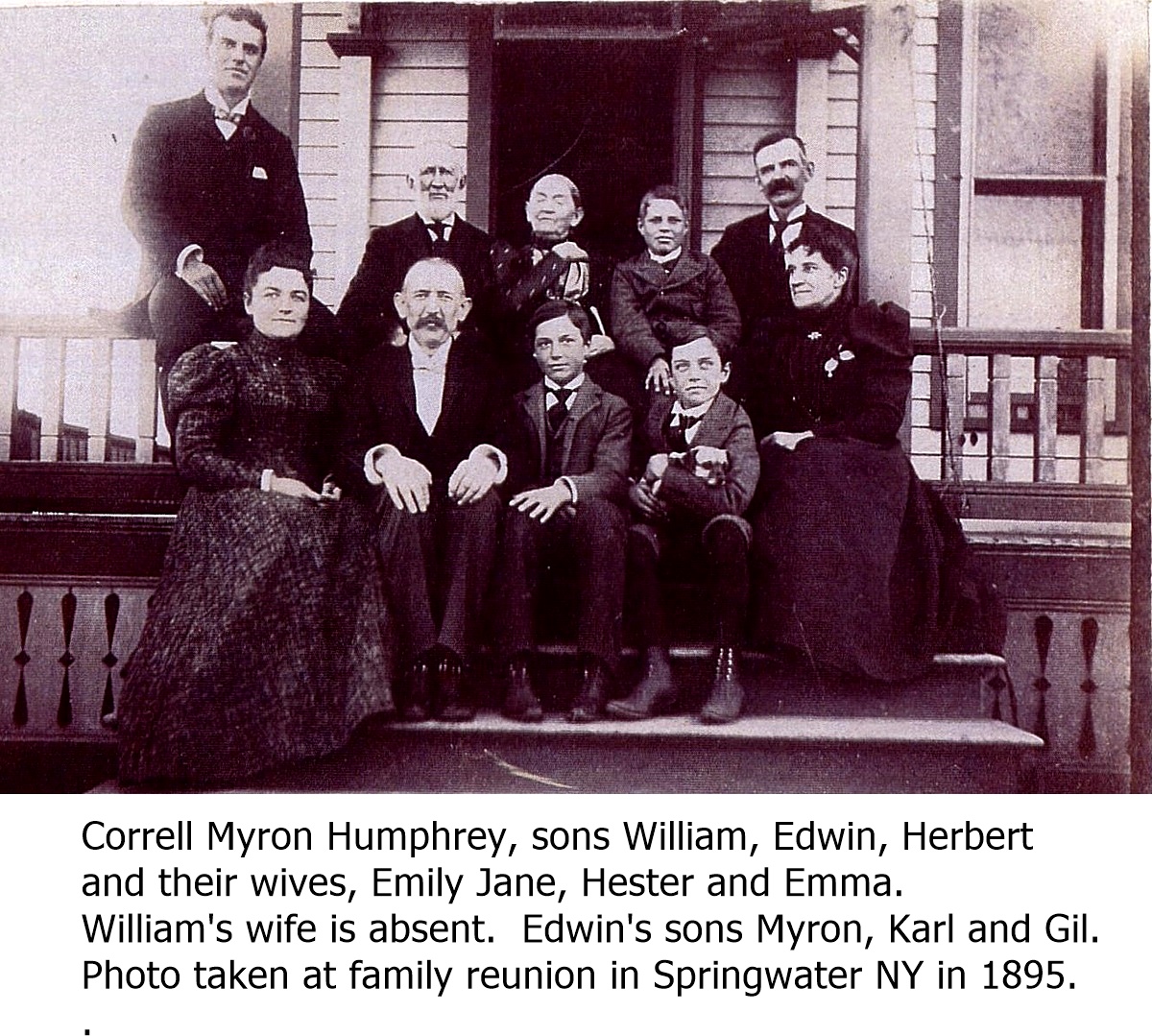In this black and white photograph from 1895, a family is gathered on the steps of a wooden porch in front of a white-paneled house with a dark brown door and windows on either side. The photo, taken at a family reunion in Springwater, New York, features men, women, and children, all dressed in formal attire. The men and boys are in black or gray suits with ties, while the women are in long black dresses with high necks and puffed shoulders.

In the front row, from left to right, sits a woman gazing forward, followed by a balding man with a long mustache. Beside him are two children, with the taller one on the left. On the far right is another woman, smiling slightly to the left. Behind her, standing on the right, is a man with a full mustache.

In the back, left to right, stand a small child, a woman with her eyes closed, an old man with a grey beard, and a young man with dark black hair, situated above the rest either standing or perched on a railing.

The names inscribed beneath the photo read: "Correll, Myron, Humphrey; sons William, Edwin, Herbert, and their wives Emily, Jane, Hester, and Emma. William's wife is absent. Edwin's sons Myron, Carl, and Gil."